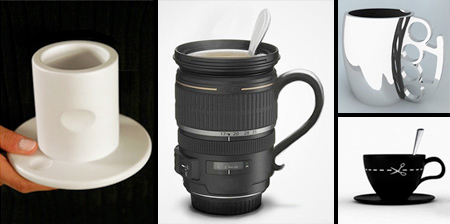The image features a set of four distinctive coffee cups displayed against a dark background. On the left, there is a photograph of a white coffee cup resting on a matching white saucer, with the entire setup slightly indented where the cup sits. To its right, a 3D-rendered coffee mug fashioned from a camera lens stands out, complete with a spoon inside, suggesting an innovative design for mixing coffee. Next to it, another 3D render showcases a metallic gray mug with a brass knuckle handle, merging functionality with a bold, edgy aesthetic. The final cup, positioned below the brass knuckle mug, is black and adorned with a graphic of scissors cutting a dotted line, adding a whimsical touch to the collection. The arrangement and creativity of these cups highlight the playful and imaginative approach to everyday coffeeware design.